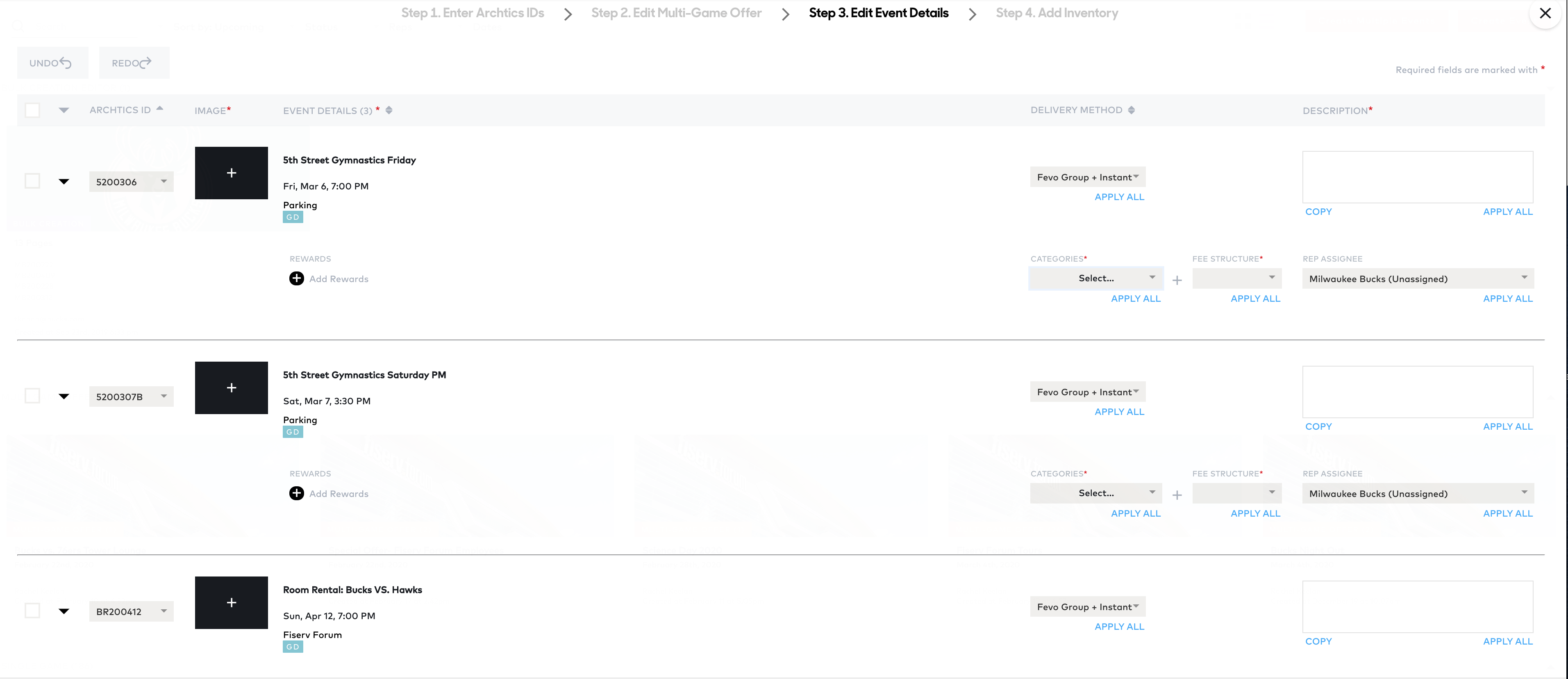The image displays a portion of a web page that contains three distinct sections. The text on the page is very small and largely unreadable, except for the tab labeled "Step 3: Edit Event Details," which is currently active. The sections are structured with multiple entries, each featuring drop-down arrows on the left side. While there are placeholders for images, none are visible. Additionally, there are more input boxes, each labeled "Apply All" in sky blue text beneath them. At the top of the page, the tabs are labeled sequentially: "Step 1: Enter Something," "Step 2: Something Game Other," "Step 3: Edit Event Details," and "Step 4: Add Inventory." The three entries within each section are separated by lines and accompanied by drop-down arrows, with additional drop-down boxes on the right-hand side, all uniformly labeled with "Apply All" beneath them.